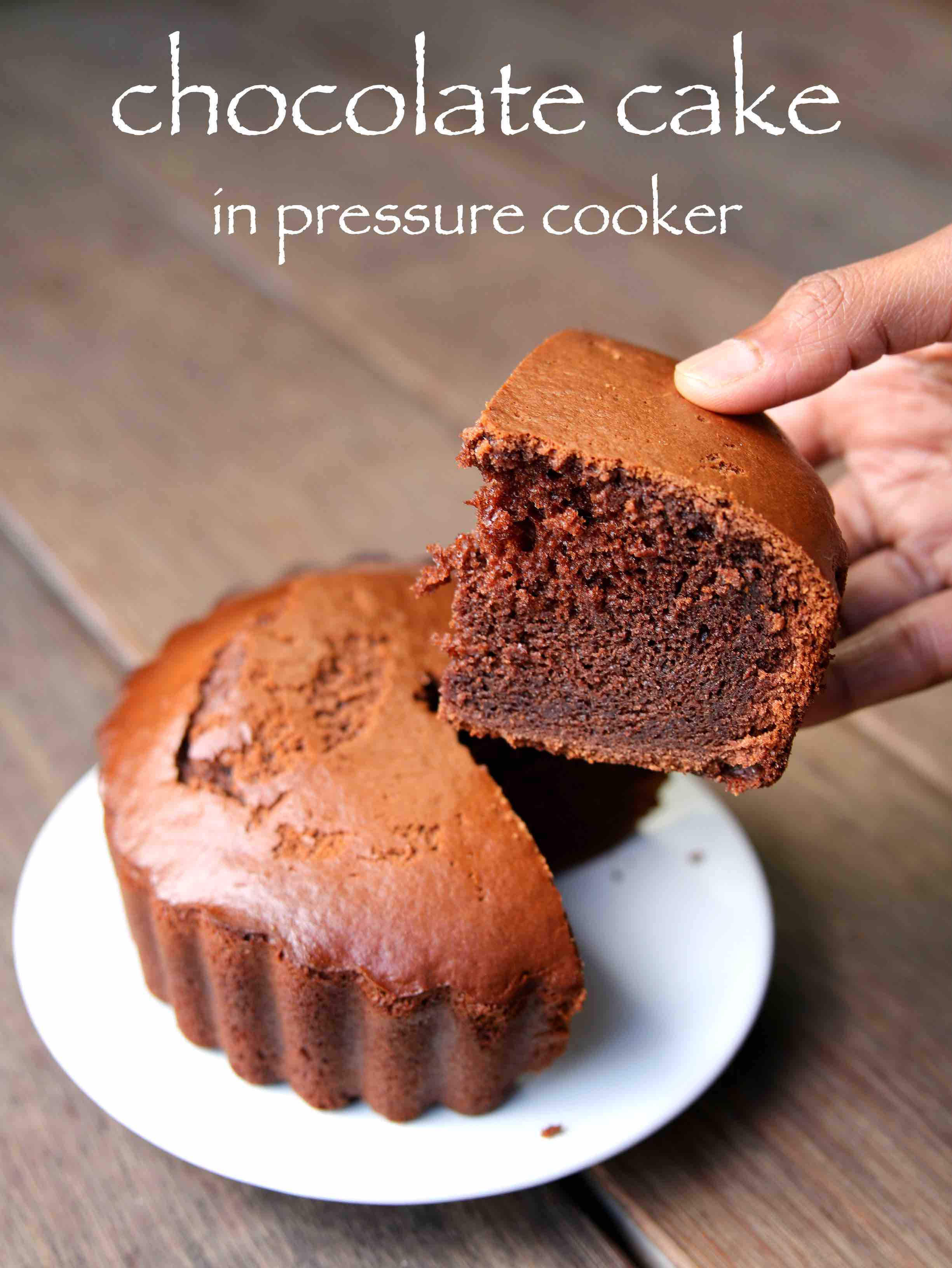In a professionally arranged and well-lit photograph, a delectable chocolate cake sits on a pristine white porcelain plate, positioned on a wide-planked, dark brown hardwood table. The circular cake has a rich, dark brown exterior with a lighter brown, almost brownie-like interior, accentuating its appetizing texture. A hand, pinkish-brown in tone, delicately holds a thick, triangular slice of the cake, lifted just above the main portion on the plate. The top of the image features the text "Chocolate Cake in Pressure Cooker" in stylish white Papyrus font, suggesting the method of preparation. The composition emphasizes neutral tones, ensuring the food remains the central focus, offering a striking visual appeal without any distracting background elements.